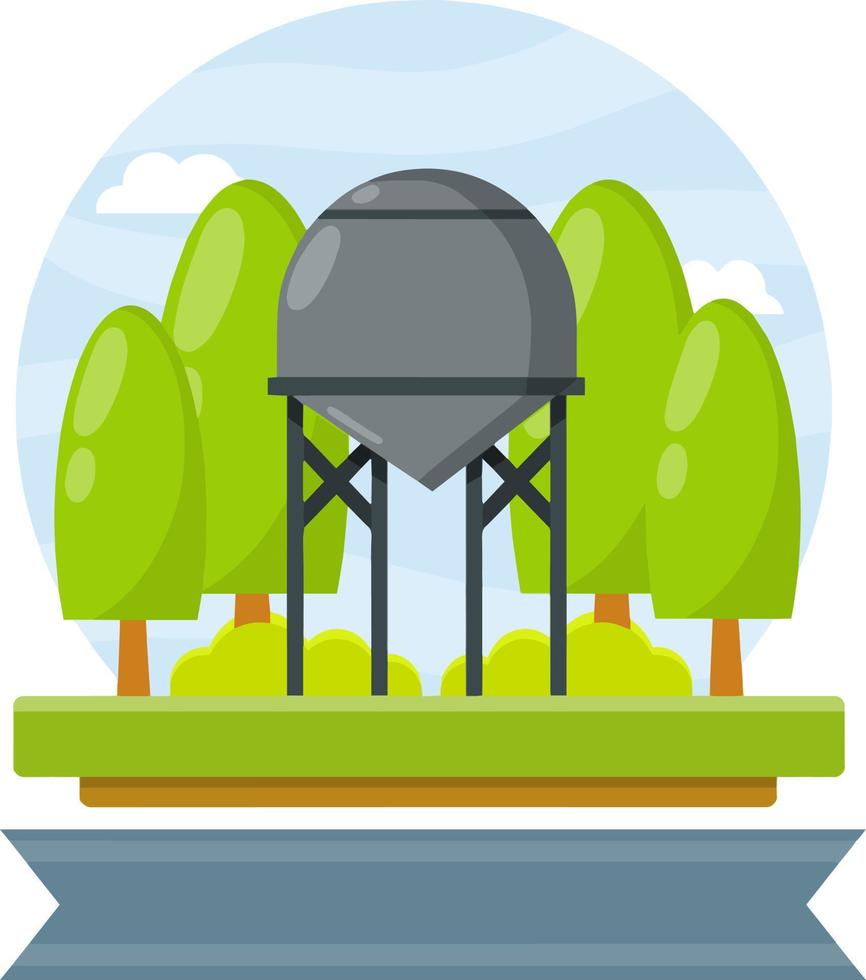The digitally-drawn image presents a cartoony depiction of a scene encapsulated within a snow globe-like structure. Inside the glass bubble, there is a central tall gray water tower, flanked by four trees arranged symmetrically—two trees on the left and two on the right. The trees, reminiscent of lollipops, have green canopies and are accompanied by two large shrubs at the base. The bottom of the globe features a greenish grass-covered surface, which transitions into a brown line denoting soil. Beneath this soil layer, there's a thick, dark blue line. The background is a clear blue sky with two white clouds. The entire design rests on a gray base platform, completing the whimsical and stylized graphic.